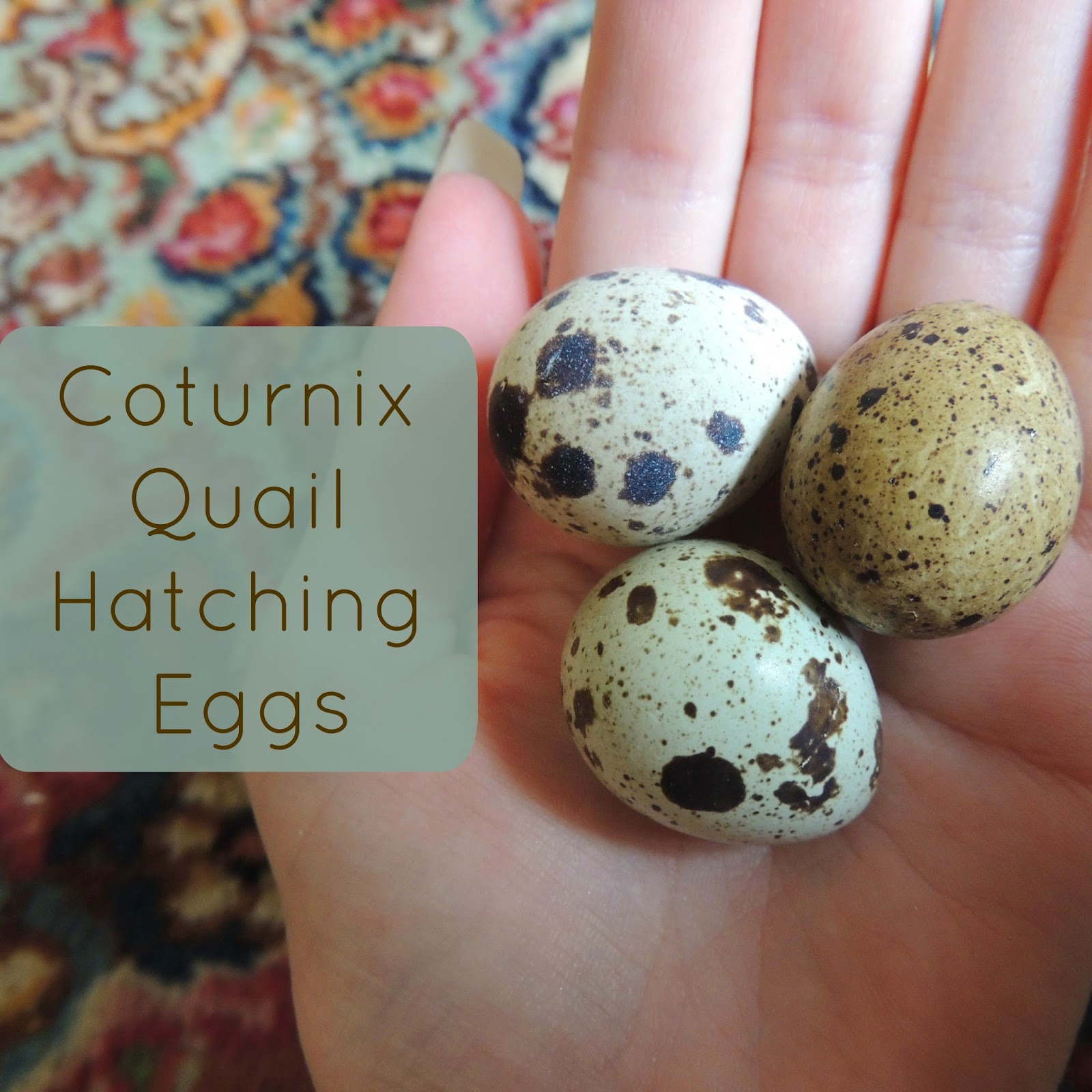The image features a close-up of a woman's hand holding three Coturnix quail hatching eggs. On the left side of the image, a text box reads "Coturnix Quail Hatching Eggs." The three eggs in the woman's hand display distinct characteristics: two eggs are primarily white with black splatter marks, resembling a speckled or dappled pattern, while the third egg, situated at the top right, is a deeper olive brown with similar dark spots. The hand holding the eggs is positioned against a background that appears to be a teal carpet with red, yellow, and blue abstract patterns, possibly flowers. The tight framing of the photo captures only the hand and the eggs, with parts of the palm and fingers extending beyond the frame. The woman's neatly manicured nails are also visible, adding to the detailed and intimate nature of the shot.